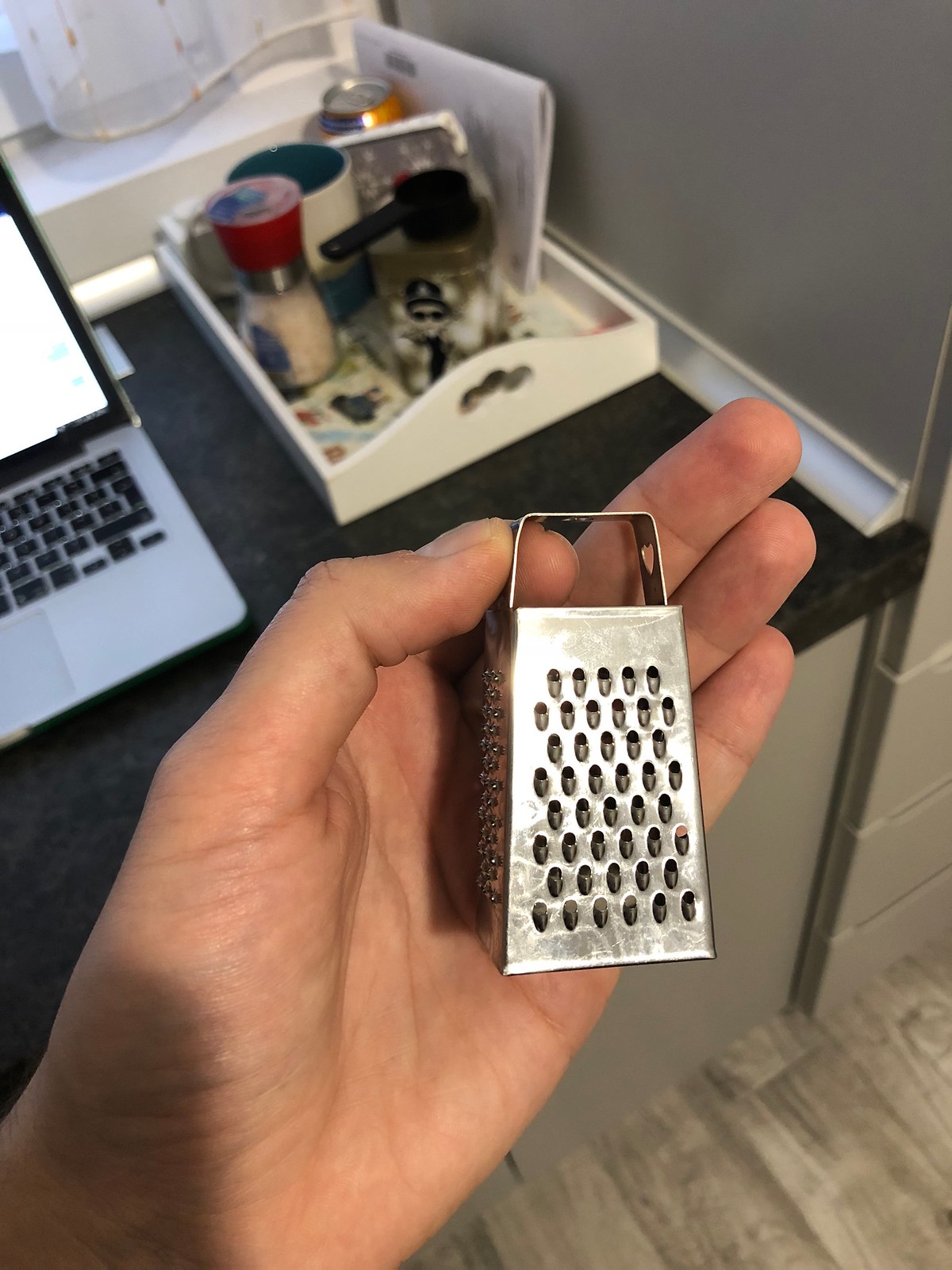The image is a color photograph depicting a pale left hand extending from the bottom left corner towards the viewer, holding a tiny metal cheese grater. The grater is clasped delicately between the thumb and forefinger, with the other fingers extended behind it. The grater's polished surface reflects light, accentuating its miniature size against the hand. In the background, there is a workspace setting with a desk. On the desk sits a partially visible laptop with a silver body and black keys, its screen blank and white. To the right of the laptop, a white open tray holds various items such as a coffee cup, potentially a coffee maker, a soda can, and possibly pamphlets or other small objects. Beyond the desk is a windowsill with a thin, sheer curtain hanging in front of a gray wall, accompanied by light gray cabinets. The scene is complemented by a light brown wooden floor, adding warmth to the otherwise cool tones of the room.